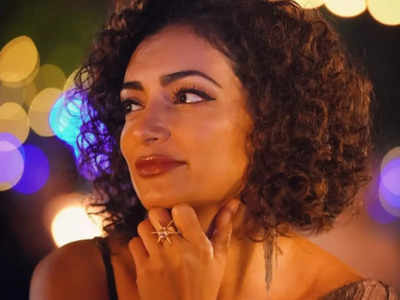The color photo features a close-up of a young woman, likely in her twenties, with light to lightly darker skin and shoulder-length, very curly, dark brown hair. She is depicted in a three-quarter view with her head slightly tilted, looking thoughtfully to the top left. Her vivid red lipstick and makeup accentuate her full, thick, black eyebrows and healthy youthful appearance. Her right hand is propped under her chin, adorned with a gold ring on her middle finger that resembles a ship's steering wheel. She wears long, dangly earrings partly obscured by her curly hair, which reaches just about her shoulders. The background is a blur of colorful, round lights, suggesting a slightly busy setting that subtly illuminates her face. She is wearing a strapless or loosely strapped dress, with the right strap casually draped over her shoulder.